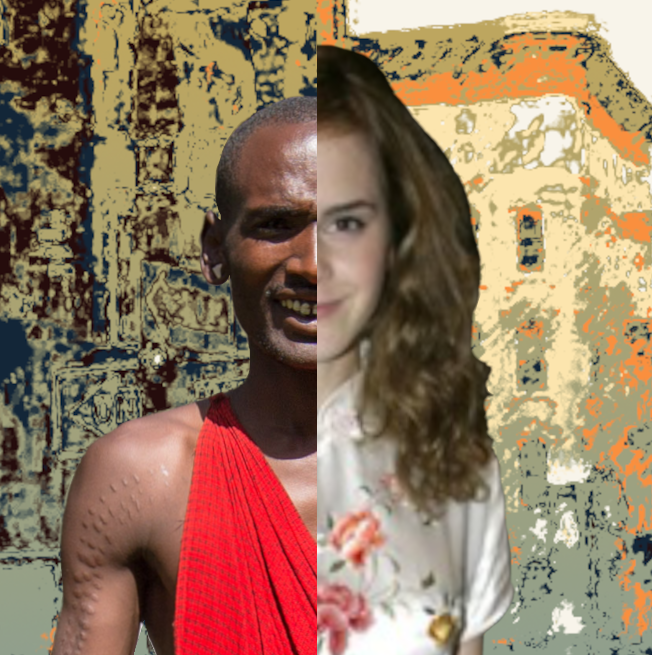The image is an intriguing composite, split vertically down the middle, juxtaposing two contrasting subjects. On the left-hand side is a Black man, presumably from an indigenous African tribe, suggested by his attire and ritualistic scars on his arm. He wears a red, sleeveless robe draped across his shoulder. His short, dark hair and distinctive ritual scarring consisting of linear marks from his shoulder down his upper arm stand out. The right-hand side features a white woman, possibly in her late teens, with chest-length wavy brown hair. She wears a white, satin-like top adorned with a floral pattern, possibly depicting roses. Both figures are smiling, and the images are aligned such that their eyes, noses, and mouths match up seamlessly, creating a visually striking split-face effect. The background of the image combines elements of an abstract drawing and a building, blending tan, brown, and blue tones to form a cohesive yet surreal setting. The combined effect emphasizes the harmonious integration of two disparate cultural representations.